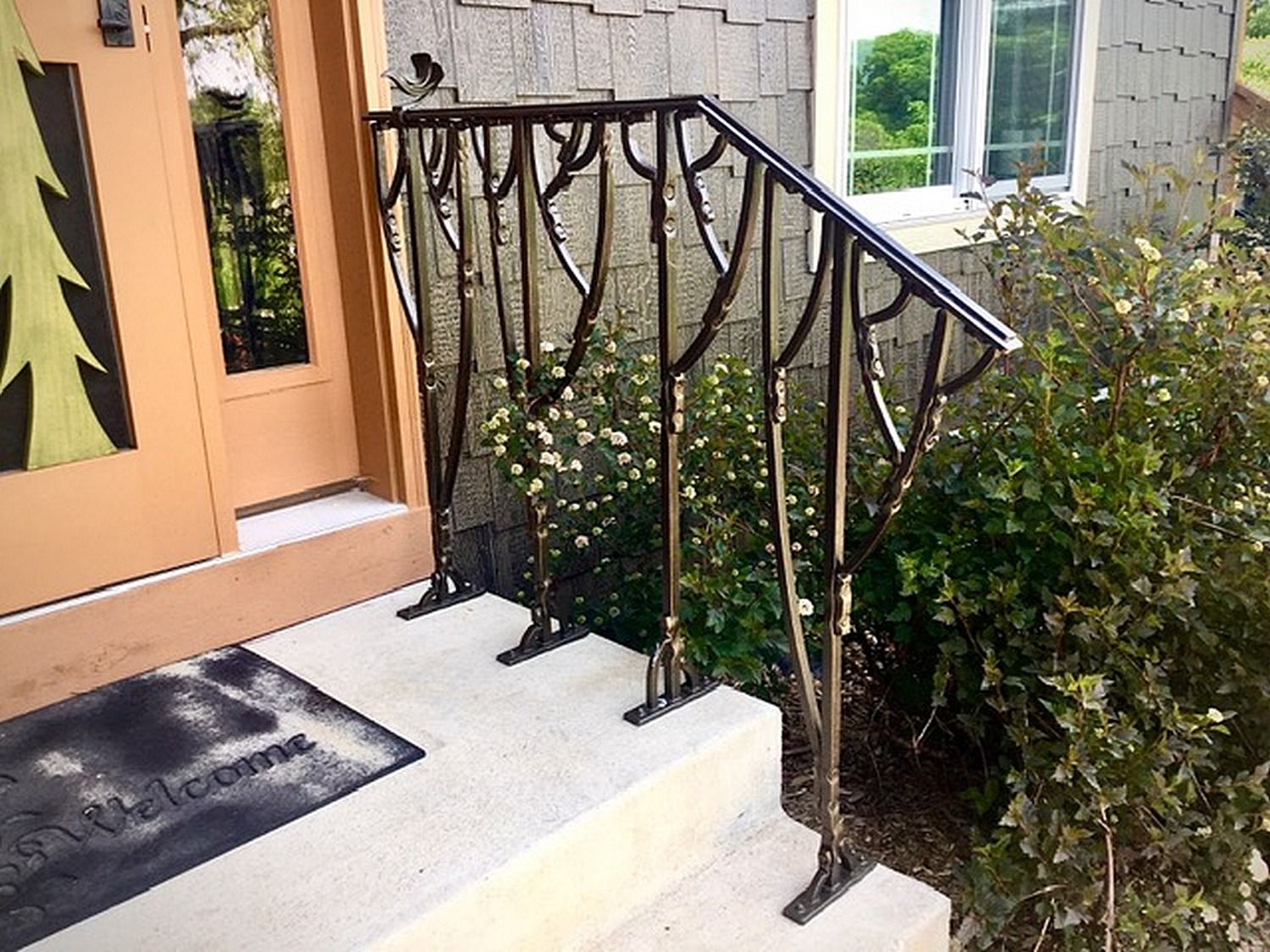The image depicts the front steps of a single-family home, primarily showcasing a metal handrail that serves as the central focal point. The handrail, made of black metal, leads up two concrete steps and features a flat top that angles down towards the right. It is supported by four square metal bars that attach to a foot on the concrete steps. Notably, a small, carved bird embellishes the top of the railing closest to the door.

In the bottom left corner, a black and white interwoven doormat rests on the concrete slab, with the word "welcome" elegantly written in cursive. This doormat appears worn in some areas, creating a mixed black and white appearance. Above the doormat is a copper-colored wooden door adorned with a silhouette of a green tree in its window, framed by a light gray paneling that covers the house exterior.

Adjacent to the steps is a garden with lush green vegetation and white flowers. Additionally, the scene includes a two-pane window with a white frame to the left of the door, further complementing the light gray siding of the house.